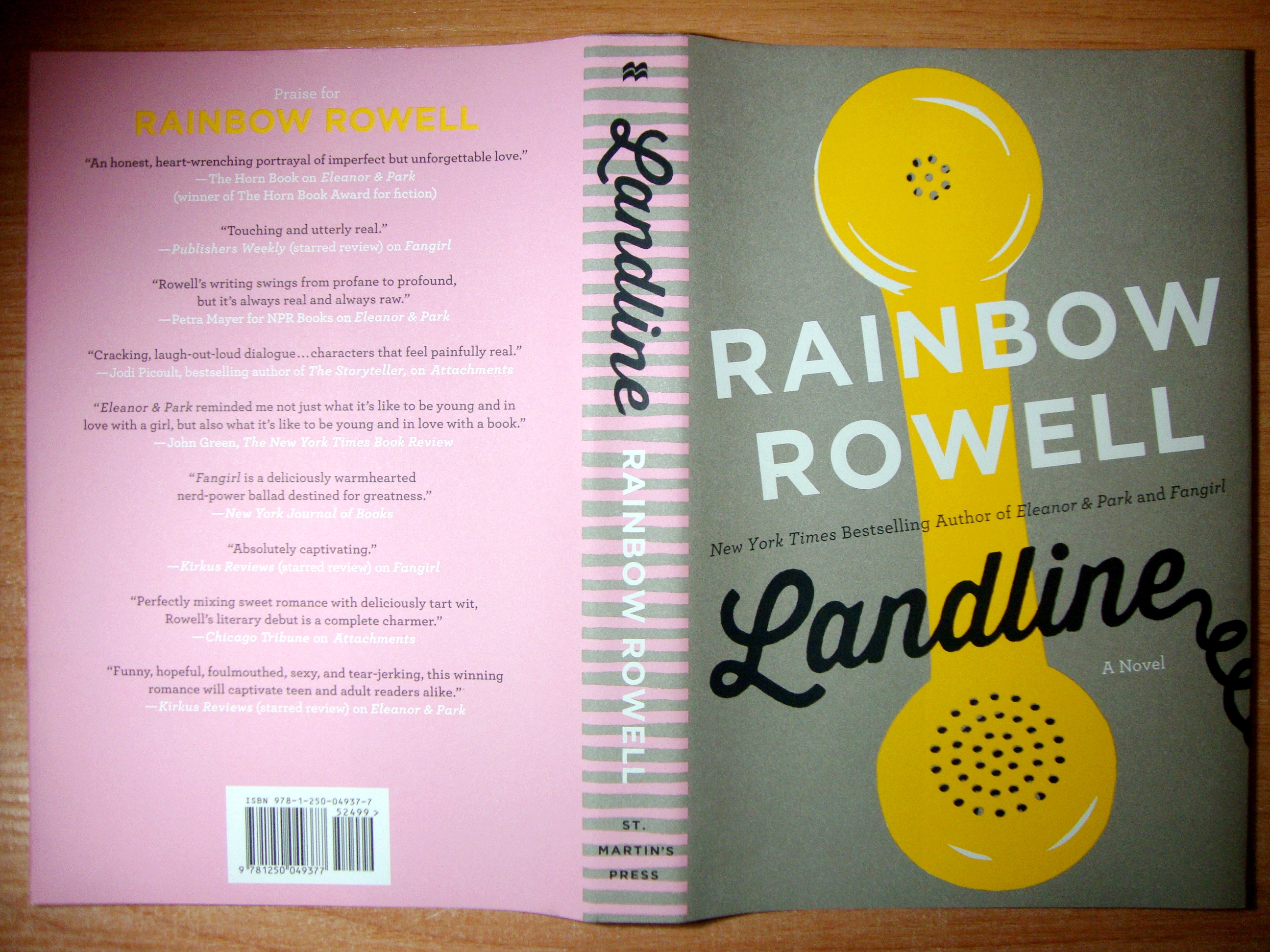The image features a book laid open, displaying both its back and front covers as well as the spine. The book, titled "Landline," is authored by Rainbow Rowell, with her name prominently displayed on the front cover in white uppercase letters. The front cover, set against a solid gray background reminiscent of concrete, showcases a bright yellow, cartoon-style corded phone. Above the phone, in a smaller gray-black font, it states "New York Times best-selling author of Eleanor and Park and Fangirl." The title "Landline" is written in large black cursive, with a playful detail where the end of the letter 'E' extends into a phone cord. 

The spine of the book, which lies in the center, features alternating pink and gray stripes with "Landline" written in black cursive and "Rainbow Rowell" in white. Below, it says "St. Martin's Press" in white.

The back cover is entirely pink with "Praise for" in white and "Rainbow Rowell" in yellow, followed by various quotes from other authors in white and black text. At the bottom of the back cover, a black and white barcode is visible.

This image is set on a grainy brown table, providing a neutral contrast to the vibrant book cover colors.